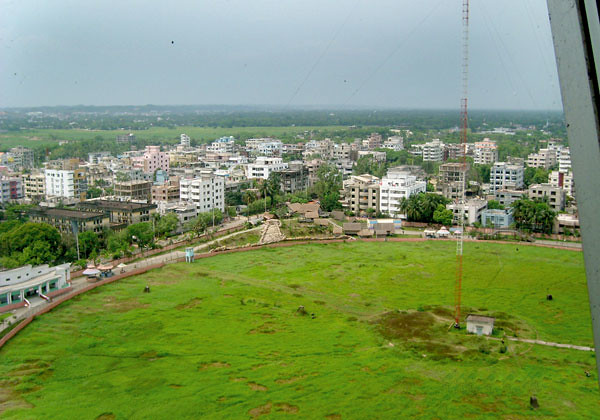This aerial view provides a sweeping overlook of a small industrial city, characterized by a mix of tall buildings, likely apartment complexes, hotels, and other residential and commercial structures. In the foreground, there's a prominent circular area of green grass, interspersed with brown dirt patches and surrounded by a low brown wall. At the center of this circle stands a tall red and white tower with alternating bands of color and wires extending downward, towering beyond the top edge of the image. Adjacent to the tower is a single-story building with a brown roof, presumably a maintenance facility. The cityscape stretches out in the midground, with a variety of white and gray buildings, some being several stories high. A pathway or road weaves through the area, connecting different sections of the city, although no vehicles are visible. The backdrop features extensive greenery and a horizon lined with trees, hinting at a somewhat rural setting despite the urban structures. The sky above is hazy, marked by a mix of bluish and gray tones, indicating a cloudy, daytime scene. The distant landscape appears to have a slight elevation, suggesting a mountainous region in the background.